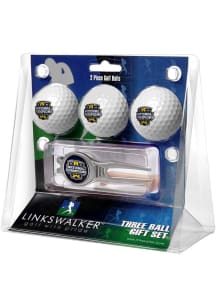This image features a packaged container of three white golf balls set against a plain white background and surface. The plastic clamshell package is presented upright, with a predominantly blue liner accented by touches of green and black. Horizontally aligned at the top of the package, the three white golf balls each showcase a logo embossed in black at their center. Beneath the golf balls, there is a rectangular tool included within the packaging.

At the bottom left of the package, a black background with bold white capital letters spells "Lynx Walker." Adjacent to this, the bottom right section features horizontal blue and green bands with thick white capital letters stating "Three Ball Gift Set."